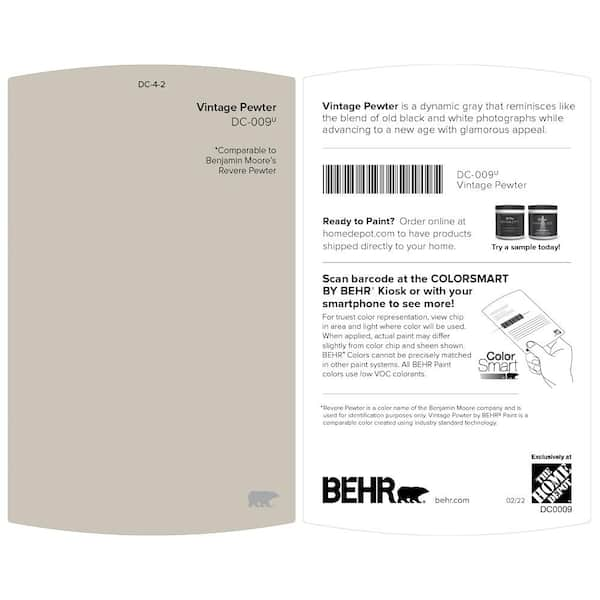The image depicts an insert for a paint product, featuring two pages, each with distinct content and formatting. The pages, slightly longer in the center than on the outer edges and rounded at the top and bottom, showcase a color swatch for Behr Paints. The left page is a delicate brown shade and presents the front of the swatch labeled "DC-009 Vintage Pewter," noted to be comparable to Benjamin Moore's Revere Pewter. The bottom right corner of this page displays the Behr logo in a slightly darker color.

The right page, which is white, is packed with information and spans across the top two-thirds with multiple lines of text and a barcode. This text describes Vintage Pewter as a dynamic gray that evokes the nostalgic blend of old black-and-white photographs while also offering a modern, glamorous appeal. It provides practical guidance, encouraging customers to order online at homedepot.com and to try a sample. The barcode can be scanned at the ColorSmart by Behr kiosk or with a smartphone for more details. The page also suggests viewing the color chip in the intended light environment, noting that actual paint may differ slightly in color and sheen. A small image in the text shows a person scanning the card, emphasizing the ease of the process. 

At the bottom of the right page, the logos of Behr and Home Depot are positioned side by side, with the Behr logo to the left and the Home Depot’s distinctive angled logo to the right, underscoring the exclusive distribution partnership.